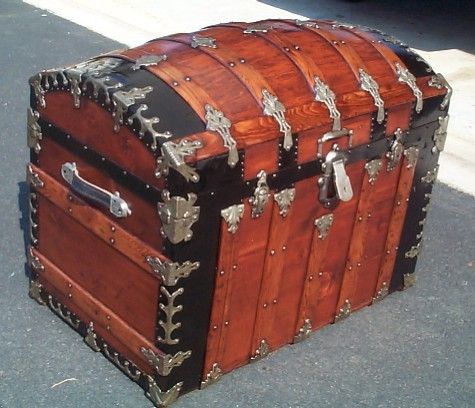The photograph captures a square, color image of an ornate, vintage wooden chest or trunk. The chest, positioned at a slight angle facing the bottom right corner of the image, stands prominently on a gray concrete surface, which suggests it is situated outdoors. The body of the chest is crafted from reddish-brown wood with horizontal wood panels, and it features vertical wooden straps reinforced with decorative, spoon-shaped silver trims. Each corner of the chest is fortified with black metal, which is further embellished with silver accents.

The top of the chest is designed in a classic humpback style, characterized by its curved, rounded lid. Black metal trim outlines the edges of the lid, echoing the design of the chest’s corners. Situated on one visible side of the chest is a silver handle with black fastenings, placed towards the top of the chest's base. A central silver latch resides at the junction of the lid and base, contributing both to the functionality and the aesthetic appeal of the piece.

The chest is large and imposing, suggesting it has the capacity to store a significant number of items. This photograph exhibits a high degree of detail, focusing solely on the chest without any other discernible background elements, emphasizing the trunk as the central subject of the image.